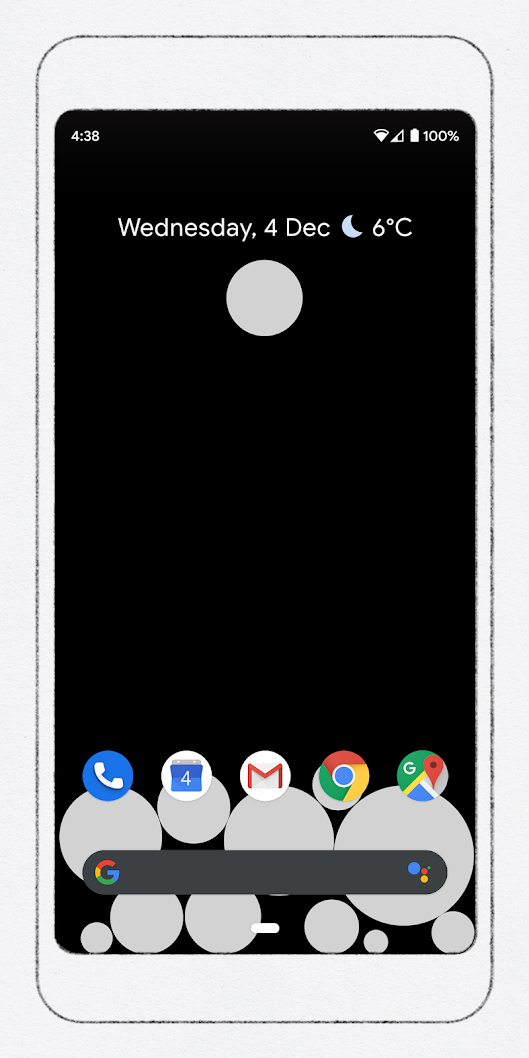This is an intricately detailed screenshot of someone's phone, overlaid onto what appears to be a hand-drawn outline of the phone itself on a white piece of paper. The outline is thin and black, resembling a pencil sketch. 

On the actual phone screen, the time displayed in the top left corner is 4:38, while the right side of the status bar shows nearly full internet connectivity bars and a battery charged to 100%. The background of the screen is predominantly black.

At the top, it reads "Wednesday, 4 DEC," indicating the date as the 4th of December. Adjacent to this text is a crescent moon icon, suggesting that the phone is possibly in Do Not Disturb mode. The current temperature is shown as 6°C, without the word Celsius fully written.

Beneath this information, there is a prominent large white circle. Approximately at the bottom quarter of the screen, several small and large white circles are clustered together. Centrally located among these circles is a long, oval-shaped dark gray bar featuring a colorful, rainbow-styled "G" for Google, alongside a small Google icon.

Above this cluster of shapes, there are icons for various commonly used applications. From left to right, these apps include the Telephone, Calendar, Gmail, Google Chrome, and Maps.